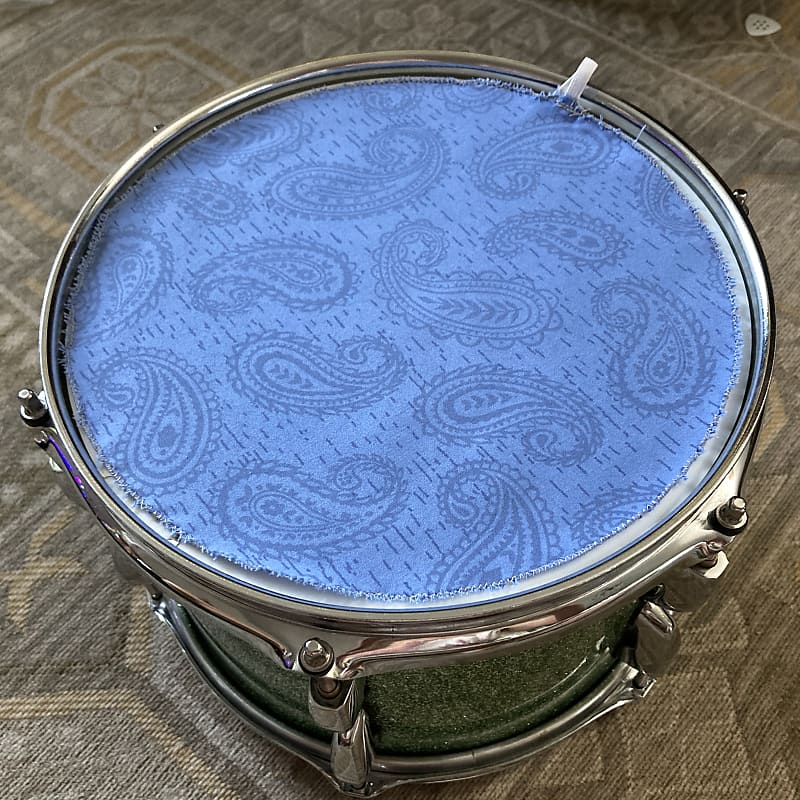The photograph captures a detailed top-down view of a metal drum, prominently positioned at the center of the image. The drum appears to be silver or metallic in color and is accentuated with reflective hardware. Draped across the drum's surface is a meticulously cut piece of fabric adorned with a light blue and dark blue paisley print, featuring frayed edges for a handcrafted appearance. The backdrop of the image showcases an ornate woven area rug with a tightly braided texture. This rug, characterized by its subdued gray and gold hues and floral patterns, enhances the intricate aesthetic of the scene. In the upper right corner of the photograph lies a guitar pick, speckled with tiny black holes, adding a subtle yet significant detail to the composition. The overall imagery highlights both the drum and the richly patterned rug with a poignant emphasis on texture and subtle color contrasts.